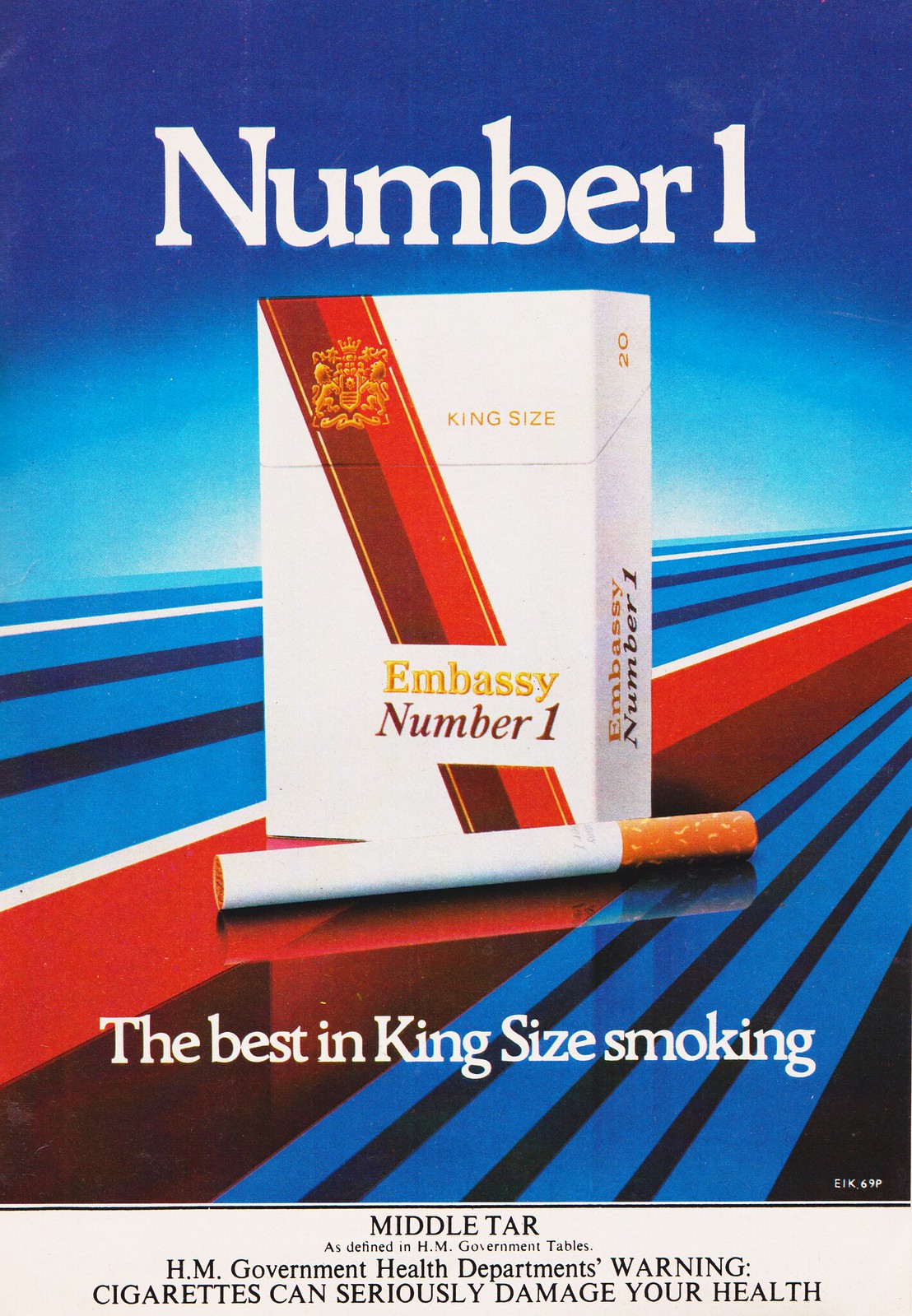The advertisement prominently features a predominantly blue background with various shades of blue, dark to light, interspersed with red, black, and white stripes running diagonally. At the top of the ad, the white text reads "Number One." The focal point in the center is a white cigarette pack branded "Kingsize Embassy No. 1," adorned with a red diagonal stripe and gold coat of arms. Just below the pack lies a single cigarette set at an angle. Beneath this, the text in white declares, "The Best in Kingsize Smoking." At the bottom, black text contains the government's health warning: "Middle tar as defined in HM government tables. HM government health department's warning, cigarettes can seriously damage your health."